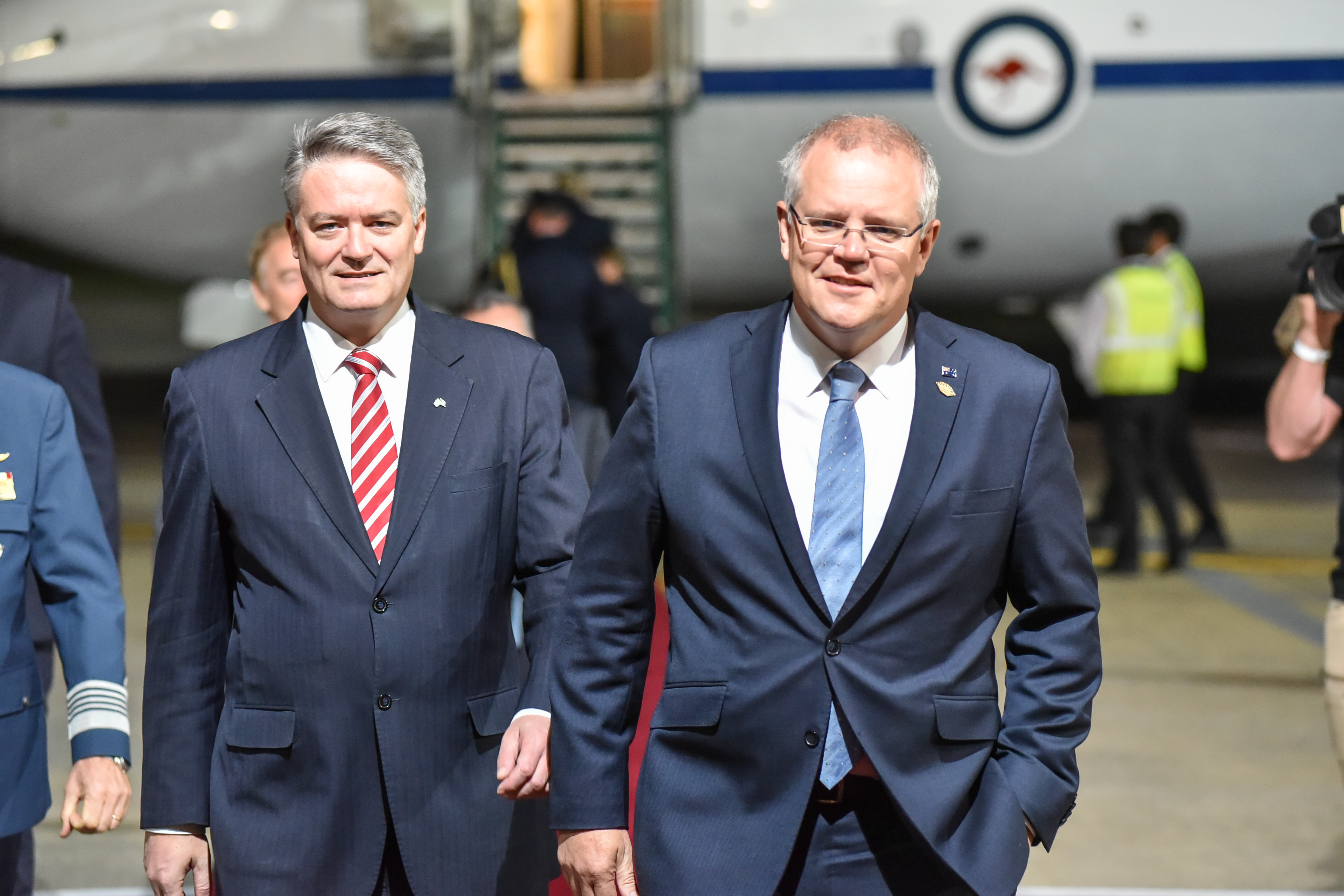The photograph captures two distinguished men, likely in their 50s or 60s, as they disembark from an airplane. Both men are dressed in navy blue business suits with white button-up shirts. The man on the left sports a red and silver diagonally striped tie and has short gray hair, while the man on the right dons a blue tie with white dots and square-framed black glasses, and is bald on top with some gray hair on the sides. They are smiling at the camera, exuding a sense of accomplishment or satisfaction. 

The background features a large airplane with a gray bottom, white top, and a distinct blue horizontal stripe running along its side. A notable circular emblem with an inner blue border and a red kangaroo is visible on the plane, indicating that it is an Australian aircraft. The plane's stairs are still down, and several personnel in neon yellow safety vests can be seen around, likely ensuring safety during the disembarkation. Additionally, a figure in military attire is partially visible on the far left, adding a layer of formality to the scene. The overall setting, combined with the men's attire and demeanor, suggests they could be politicians or officials arriving for an important event.